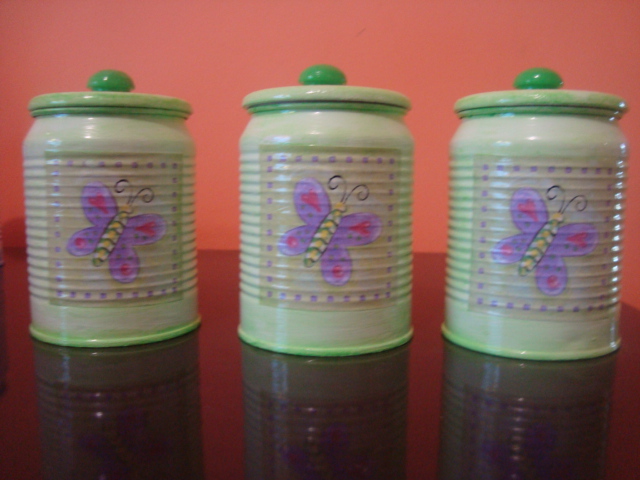The image captures a well-lit indoor scene featuring three identical ceramic canisters arranged symmetrically on a shiny, reddish-brown countertop. The reflective surface beautifully mirrors the canisters, enhancing the visual appeal. These light evergreen canisters have matching lids with darker green knobs for easy handling. The background is a dark peach, almost orangish-red wall that adds warmth to the setting. Each canister showcases a charming, child-like illustration of a purple butterfly encased within a cream-colored rectangular frame. The butterfly’s wings are adorned with red hearts in the upper sections and red dots in the lower sections. Its yellow body, detailed with black stripes, is complemented by black, slightly curved antennas. Surrounding the butterfly are delicate light purple dots that accentuate the whimsical design. The green rims around the top and bottom of the canisters add an elegant touch, making them perfect for storing kitchen essentials like flour, sugar, or coffee.